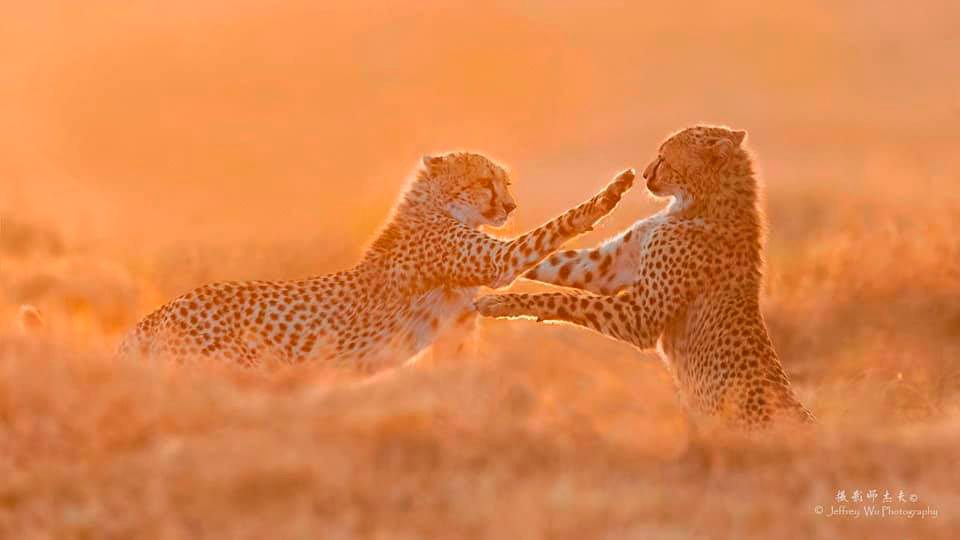The image portrays two leopards, though initially mistaken by some for jaguars or cheetahs, standing in the center of the frame bathed in an omnipresent orange tinge that blurs the surroundings. Both leopards appear to be playfully interacting; the one on the left, with its right paw extended, seems to be reaching for the leopard on the right. This second leopard, facing left, is almost upright on its hind legs, with paws positioned as if touching the other leopard's shoulder and chest. Beneath them, hints of brush or grass are visible, though these too are suffused with the intense orange light, blending into yellow and green shades. The overall scene is somewhat indistinct except for the leopards, accentuating their playful interaction within this vivid yet blurry environment. In the bottom right corner, the image is marked with Asian characters followed by the text "Jeffrey Wu Photography."